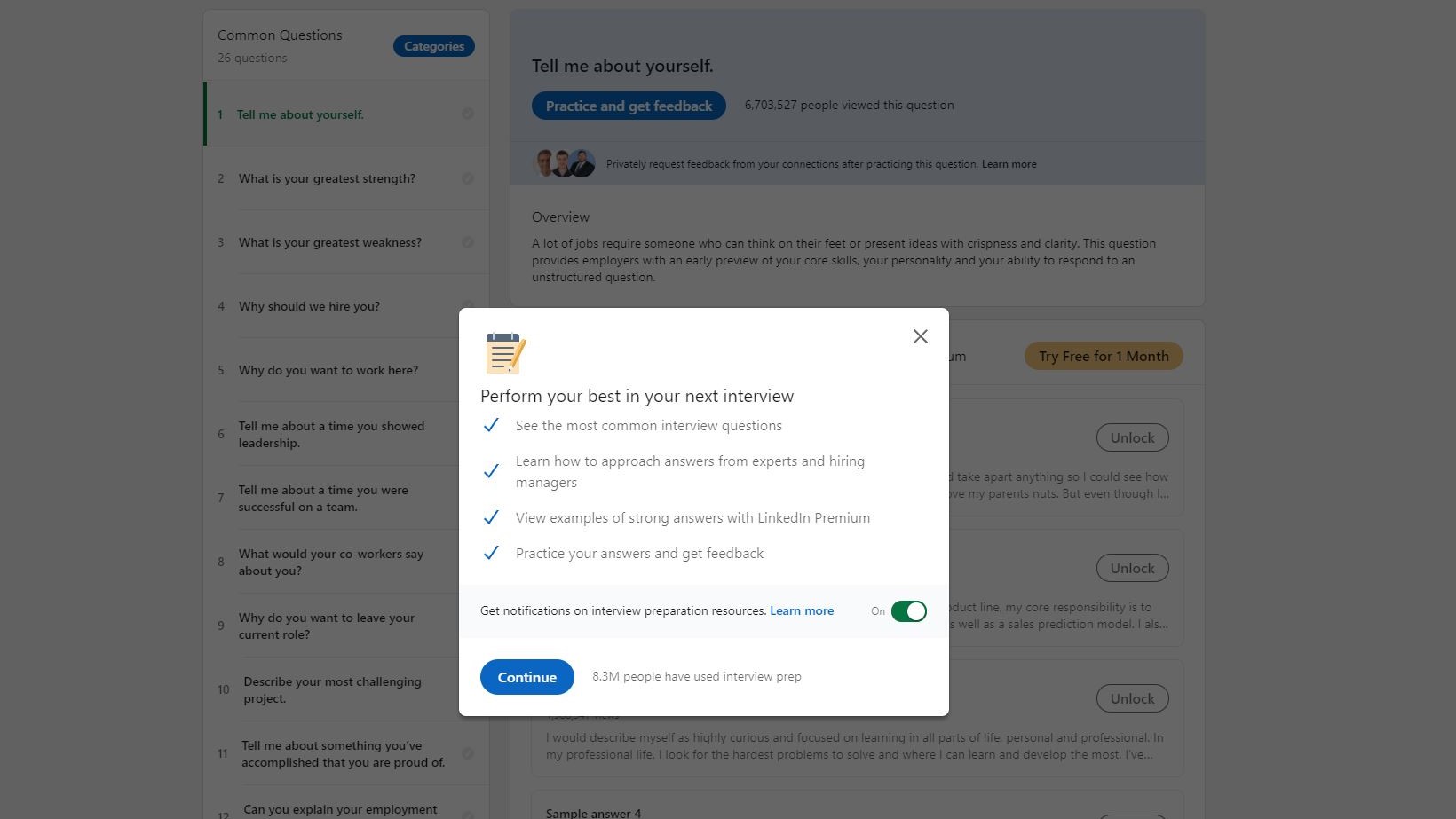**Screenshot of LinkedIn Interview Prep Tool with Pop-Up Window**

This image is a screenshot of the LinkedIn Interview Prep tool, currently featuring a pop-up window that grays out the background. The pop-up displays a message encouraging users to "Perform your best in your next interview" and offers a series of interactive options. These options include:

- Viewing the most common interview questions.
- Learning how to approach answers with insights from experts and hiring managers.
- Accessing examples of strong answers, which are enhanced with LinkedIn Premium.
- Practicing answers and receiving feedback.
- Getting notifications on additional interview preparation resources.

The pop-up features a toggle button, which is currently switched on, along with a prominent blue "Continue" button. A small gray text underlines the popularity of the tool, noting that "8.3 million people have used interview prep."

In the grayed-out background, we can see a list of common interview questions typically found on the LinkedIn Interview Prep page, including:
- "Tell me about yourself."
- "What is your greatest strength?"
- "What is your greatest weakness?"
- "Why should we hire you?"
- "Why do you want to work here?"
- "Tell me about a time you showed leadership."
- "Tell me about a time you were successful on a team."
- "What would your co-workers say about you?"
- "Why do you want to leave your current role?"
- "Describe your most challenging project."
- "Tell me about something you've accomplished that you're proud of."

The screenshot effectively illustrates LinkedIn's resources aimed at helping users prepare for job interviews by providing extensive guidance and examples.